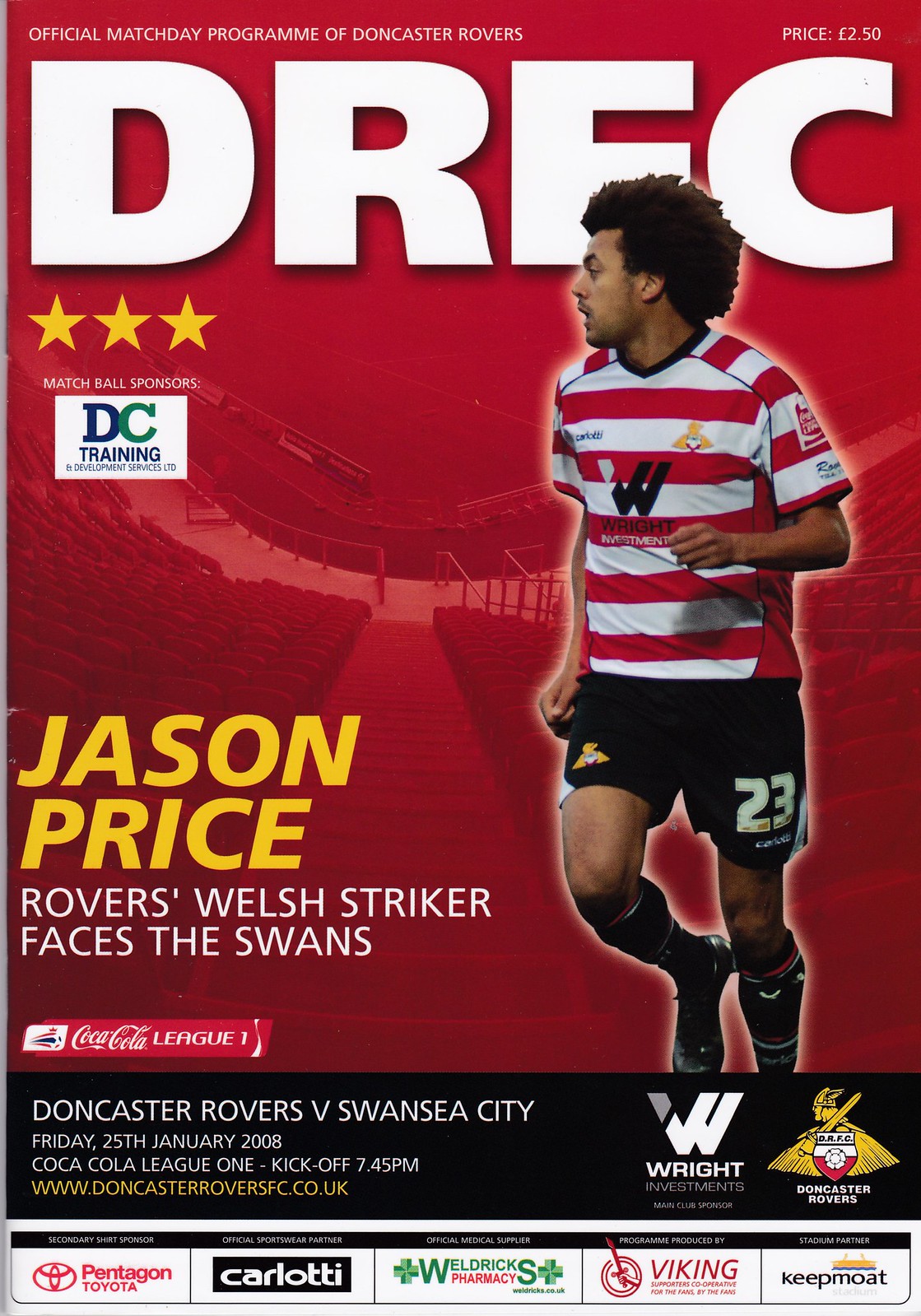The image is a magazine cover, specifically the official match day program for the Doncaster Rovers. The cover features a striking red background with a stadium bleacher view. In large, bold white letters at the top, it reads "DRFC." Below this, there are three small yellow stars and a tiny white square with some letters in it. The top left corner also states "Official Match Day Program of Doncaster Rovers," while the top right corner shows the price, £2.50.

Prominently featured on the right side of the cover is a soccer player. He appears to be a black man with poofy, curly dark hair, wearing a red and white striped jersey with the number 23, black shorts, black socks, and soccer sneakers. His stance suggests he's about to run, with one knee bent and an arm partially folded.

On the left side of the cover, in bold yellow letters, it says "Jason Price," followed by the white text "Rovers Welsh Striker Faces the Swans." There is a small Coca-Cola banner, along with additional advertisements like Toyota and Viking scattered around. At the bottom, a black bar provides match details: "Doncaster Rovers vs. Swansea City."